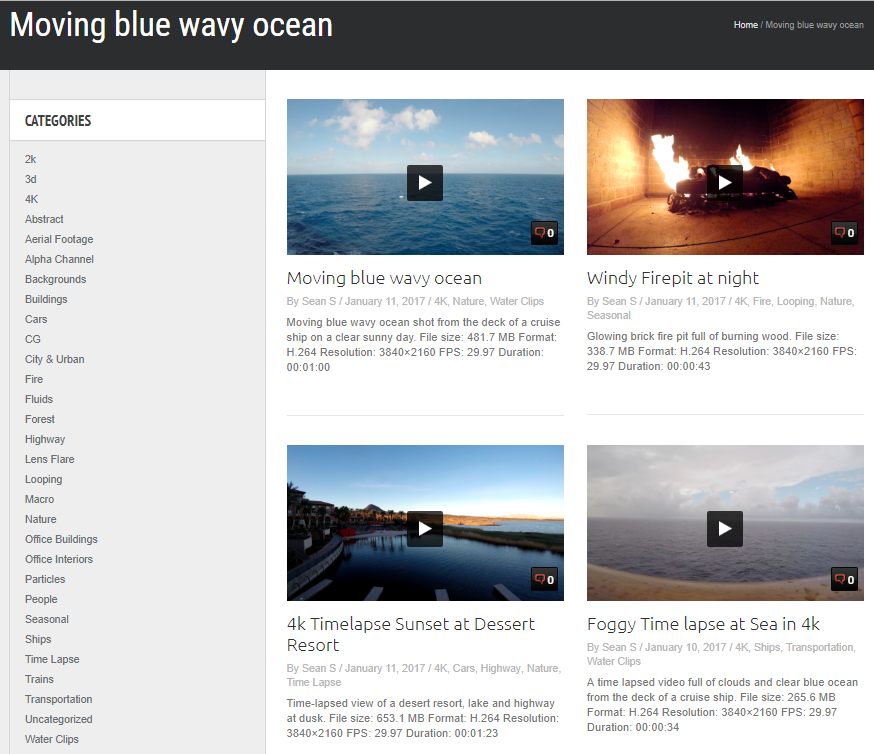This screenshot is from a website featuring a black menu bar at the top and a gray sidebar listing categories on the left-hand side. The main content area showcases four videos arranged in a 2x2 grid, each accompanied by a brief description. The black menu bar at the top displays the text "Moving Blue Wavy Ocean" in white, with a breadcrumb navigation on the right reading "Home / Moving Blue Wavy Ocean."
 
The left-hand sidebar categorizes content with labels including 2K, 3D, 4K, Abstract, Aerial Footage, Apple Channel, Backgrounds, Buildings, Cars, CG, City and Urban, Fire, Fluids, Forest, Highway, Lens Flare, Looping Macro, Nature, Office Buildings, Office Interiors, among others.

The four videos, displayed in a rectangular grid, include:
1. **Moving Blue Wavy Ocean** - Situated at the top-left.
2. **Windy Fireplace at Night** - Located at the top-right.
3. **4K Time-lapse Sunset at Desert Resort** - Positioned at the bottom-left.
4. **Foggy Time-lapse at Sea in 4K** - Found at the bottom-right.